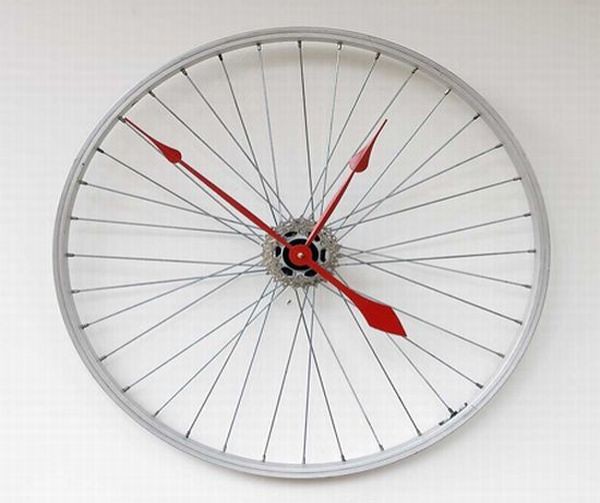This image features an intriguing clock crafted from a bicycle wheel hub. The clock retains the wheel's original spokes, giving it a distinctive and industrial aesthetic. The center is accented with a segment of bicycle chain, adding to its unique design. The clock does not feature traditional numbers, emphasizing its minimalist style. Its bold and vivid red hour, minute, and second hands stand out sharply against the background. The backdrop is primarily white but has a subtle grid texture, which adds a touch of depth to the overall composition without being overly distracting. The clock appears to be mounted against this textured white surface, making it the focal point of the image.